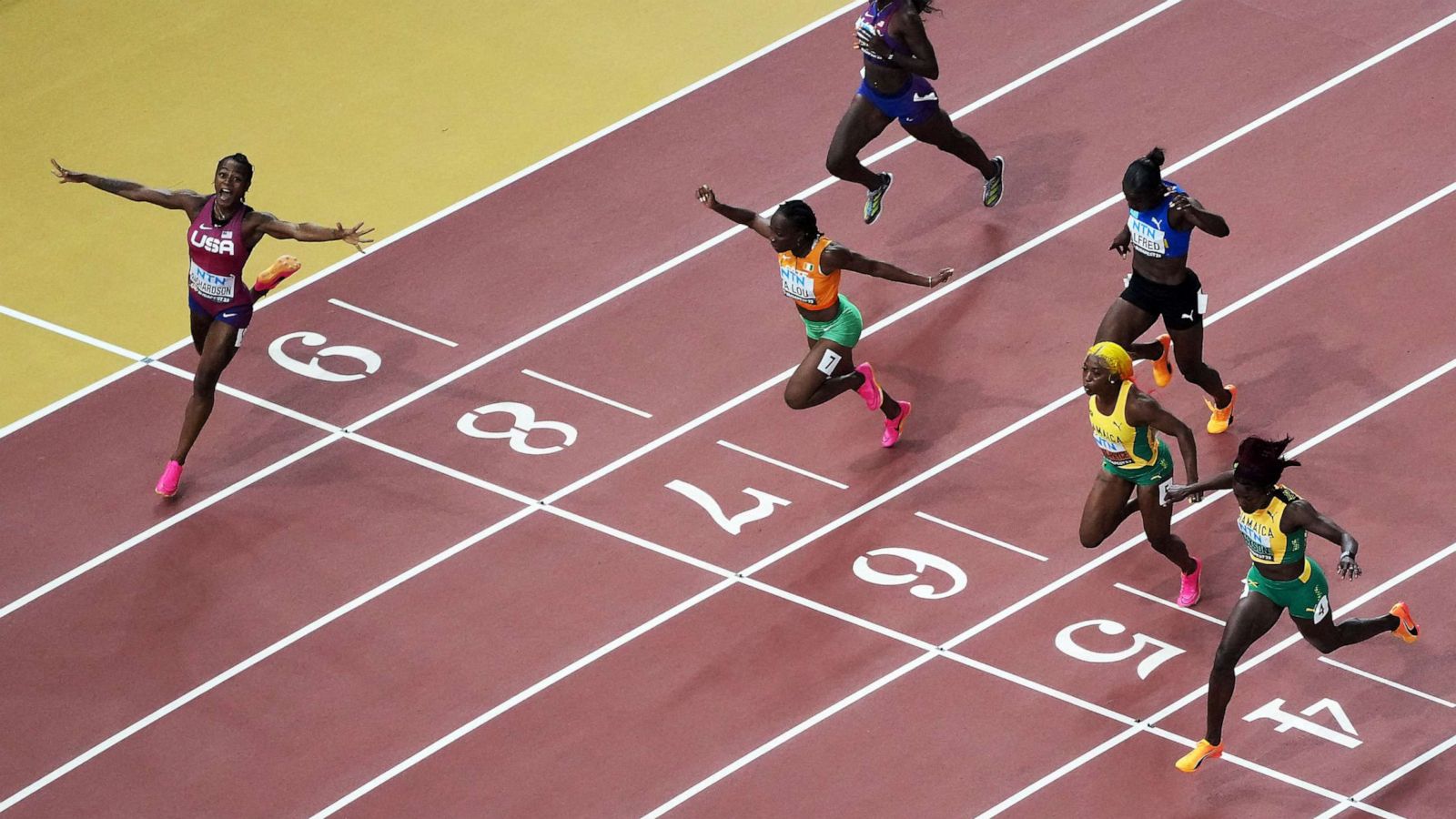This photograph captures the climactic finish of a women's sprinting race, featuring six runners on a red track numbered 4 through 9, with a contrasting solid yellow surface beyond. The jubilant winner, an African-American woman in lane 9, clad in a pinkish-red leotard emblazoned with "USA," celebrates triumphantly. She propels herself forward, arms outstretched in victory, with her right leg kicked back, revealing her pink shoes. Her beaming smile underscores her achievement. 

In stark contrast, the runner in lane 8 trails furthest behind, visible only from the neck down. Familiar faces from the world of sprinting populate the other lanes. Ta Lu in lane 7 dons green tight shorts and an orange midriff-baring top. Lane 5 hosts a renowned Jamaican sprinter in green and yellow, and another Jamaican sprinter, similarly attired, occupies lane 4. Each runner's position and demeanor reflect the race's intensity and competitive spirit, painting a vivid picture of dedication and exhilaration.